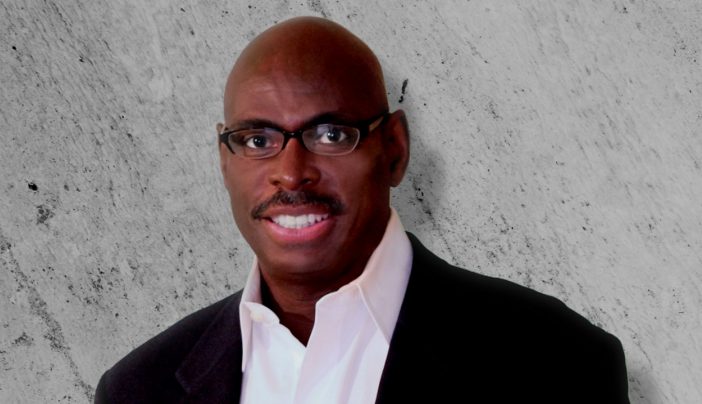This is a detailed portrait of an African-American man, portrayed from his head to about his chest. He has a bald head, black glasses, and a black mustache. His smile reveals very white teeth, giving him a kind and approachable appearance. He is dressed in a black tuxedo jacket over a white collared button-up shirt. The background features a marble-like texture, light in color with black and gray specks and streaks, providing a sophisticated backdrop. The man is facing directly at the camera with his dark brown eyes, suggesting a professional, possibly business-related setting.